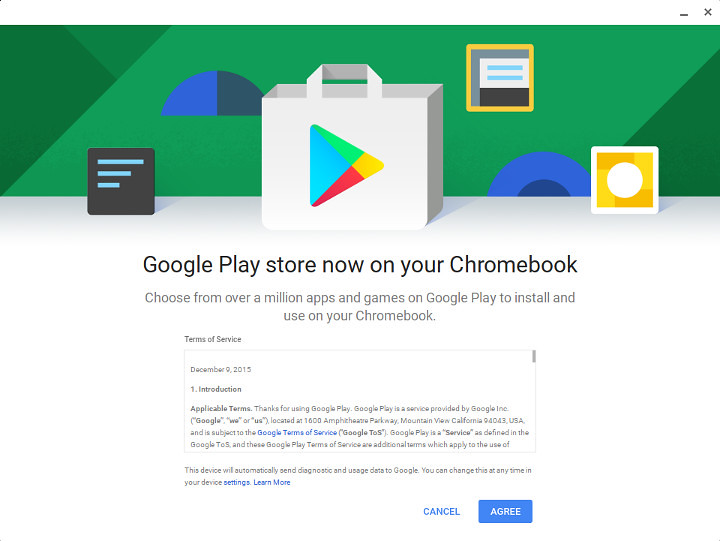This is a screenshot of a notification window typically seen on a computer, likely describing the integration of the Google Play Store with a Chromebook. The window has a standard layout with a minimize button (represented by a minus symbol) and a close button (represented by an X) located at the top-right corner. Below this top bar, the background is green, featuring an icon that resembles a text document, characterized by blue lines of decreasing length stacked from top to bottom against a black block. Adjacent to this icon is a half-circle, split into two halves: one half is blue and the other half is black.

Centrally positioned in the green background is the Google Play Store logo, depicted as a multi-colored play button within a shopping bag, incorporating yellow, green, red, and blue colors. Beneath this logo, in bold black text, the message reads: "Google Play Store now on your Chromebook." Following this, in smaller gray text, it states: "Choose from over a million apps and games on Google Play to install and use on your Chromebook."

At the bottom of the window, there is a section for the Terms of Service, accompanied by a scroll bar for additional navigation. Positioned at the bottom-right corner are two options, "Cancel" and "Agree," each placed against a dark blue background.